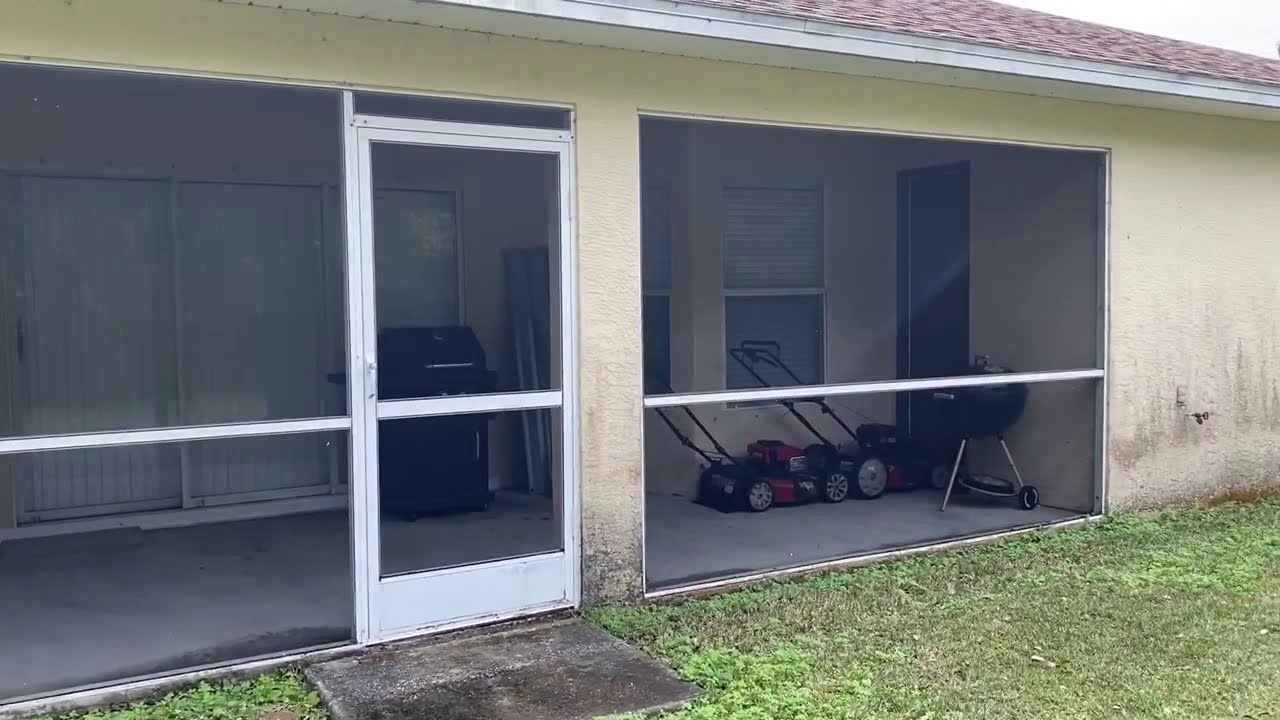The image features the exterior of a single-story house with cream-colored, slightly grimy walls and a red-tiled roof. The house appears to have both a partially outdoor area and a partially indoor setting, particularly a large screened-in porch, which serves as a patio. The porch is enclosed with two large screen windows and a white frame screen door, positioned in front of a small cement block. 

Inside the screened porch, there is a concrete floor, and the interior contains a variety of items. Notably, there are two push lawnmowers, one red and one black, positioned in front of two white framed glass windows. To the right of the lawnmowers, a black charcoal grill leans against a wall, while on the left side, a black propane grill sits in front of a large glass sliding patio door with white blinds. An opened door is also visible beside the charcoal grill. 

The yard in front of the house has a green but slightly neglected lawn, with patches of cut but somewhat dead grass. The overall scene conveys a sense of casual storage and utility within the semi-enclosed porch area.